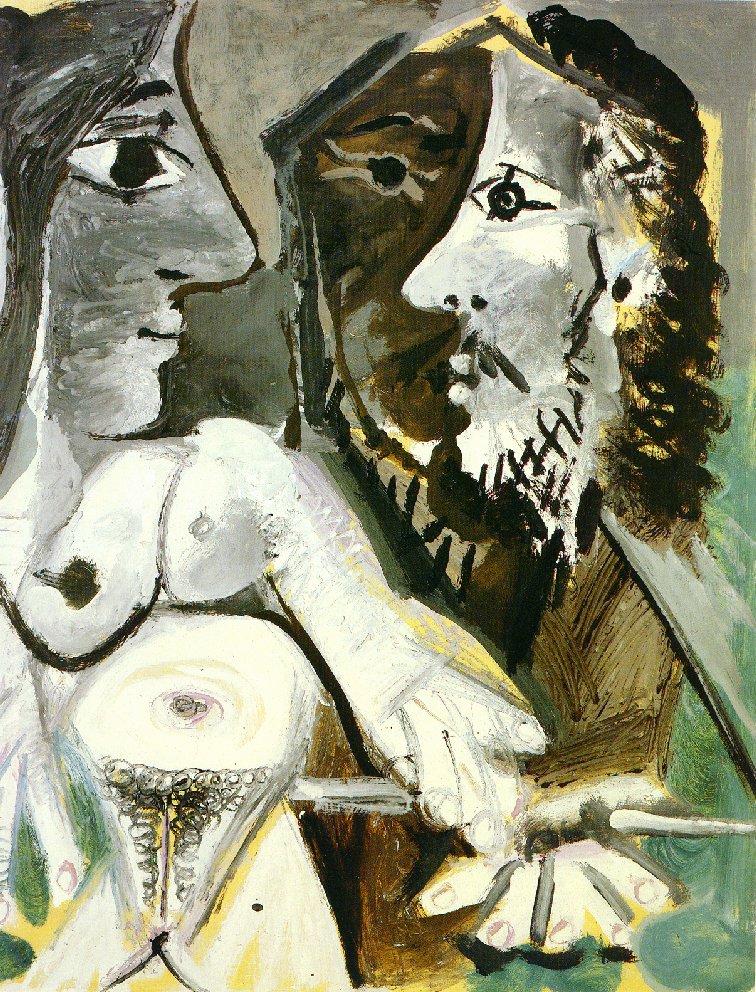This painting, resembling a Picasso-esque style, features a complex and intriguing composition of three human figures. Dominantly portrayed in acrylic, the central focus is on a woman and a man, both depicted with deformed and fragmented facial features. On the left, the naked woman with black hair is positioned closer to the viewer, her broad smile and black eyes directed towards the right. She is rendered in shades of grey, black, beige, and white, with her body exhibiting detailed impressions of her breasts, stomach, navel, and pubic area. 

To her right, a man with curly black hair, a mustache, and beard gazes back at her. His face is divided into a brown left half and a white right half, and notably lacks a mouth. The man's depiction features more vibrant colors, including yellow and beige, adding to the dynamic contrast of the painting.

An optical illusion creates the appearance of a third, mask-like face between the man and woman. This face, appearing in green tones, seamlessly blends into the overall composition, contributing to the painting's surreal and multifaceted visual narrative. The background, painted in hues of olive, clay, and green, further enhances the artwork's vivid and somewhat disorienting aesthetic.